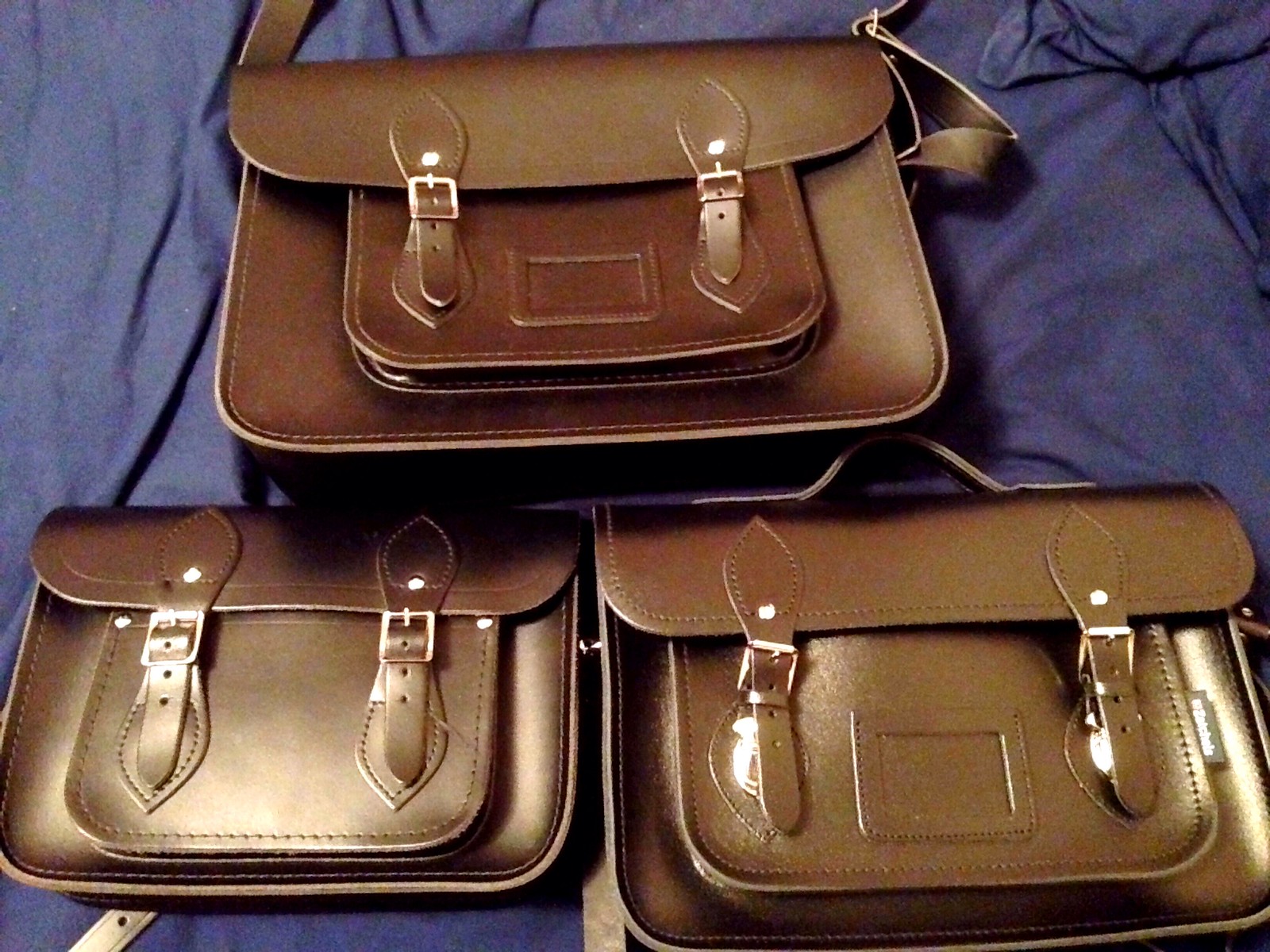This is a color photograph of three brown handbags arranged on a dark, bluish-purple fabric, which appears to be a bedsheet. All three handbags are made of a shiny, leather-like material and feature a flap over the top, secured by two buckles. Each bag also has a small front pocket beneath the flap. The handbags are positioned with two at the bottom, placed side-by-side, and one on top, slightly centered above them. While the handbags share the same design, the one at the top appears to be the largest. A portion of the strap, which matches the brown color of the bags, is visible on the right side of the top handbag. The edges of all three handbags are touching in the middle, creating a cohesive display.